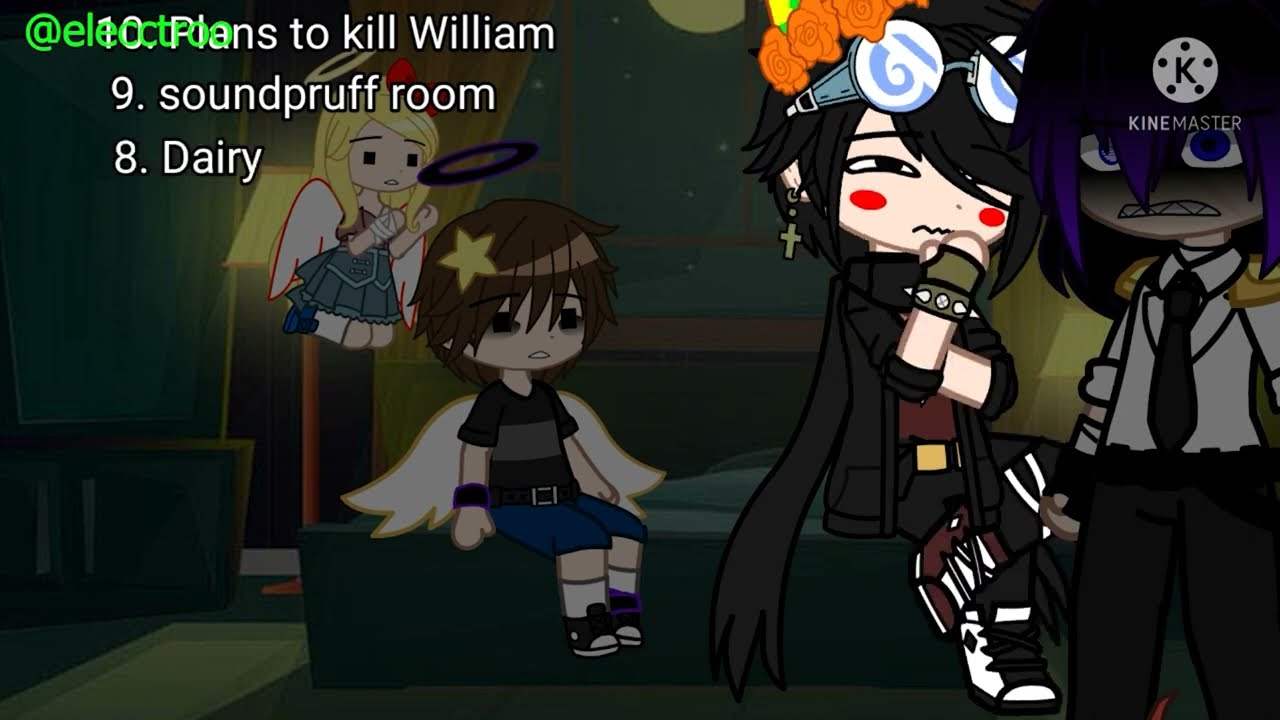In this detailed image, we see a scene populated by 2D cartoon characters, seemingly from a video game or an animated series. The setting appears to be a room full of people, most of whom are faded out to emphasize the primary characters. In the top left corner of the screen, text in green reads "AT Electro", followed by a list of plans from 10 to 8, written in white letters: "10. Plans to kill William, 9. Soundproof room, 8. Derry." The right side of the image includes the words "KineMaster" in white, accompanied by a white circle with five dots.

On the left side of the image, there is a blonde-haired angel-like character with a golden halo, white wings, and a greenish or gray dress, flying in the air. Below her, seated on a bed, is a boy angel with dark brown hair, a yellow star on his head, a blue halo, and dark eyes. He is wearing a black shirt with a gray stripe, blue jeans, a black belt, white socks, blue and white shoes, and a black watch. His expression appears worried, with a downturned mouth and large eyes.

To the right, we encounter a more intimidating character with black hair partially covering her left eye, donned with red circles on her cheeks. She has a cross earring, goofy glasses with swirly lenses on her head, and is dressed in a dark outfit consisting of an all-black ensemble, a brown undershirt or gold pants, and a sort of cape. Completing the scene, another scary-looking figure stands to her right, characterized by blue hair, purplish eyes, sharp teeth, and a scowling expression. This figure is dressed in a white uniform with a chain connecting the shoulder pads, a dark blue or black tie, and black pants. The room features a yellow-lit lamp with a brown base, a dark green floor, a dark green bed, and a white mat at the doorway, suggesting a bedroom setting.